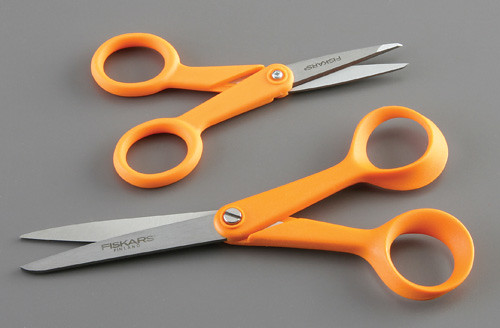A photographic image captures two pairs of scissors placed on a gray surface that appears to be a table or a platform. The scissors are positioned opposite each other, with the smaller pair on top and the larger pair on the bottom. The smaller pair has its blades pointing toward the top right corner of the image, while the larger pair points toward the bottom left. Both pairs of scissors have bright orange handles with large holes for gripping, and they share a similar design. Inscribed on the grayish steel blades of both pairs is the brand name "Fiskars," accompanied by additional text that is too small to decipher. Each pair of scissors is slightly open, revealing a silver flat-headed screw that fastens the blades and handles together.